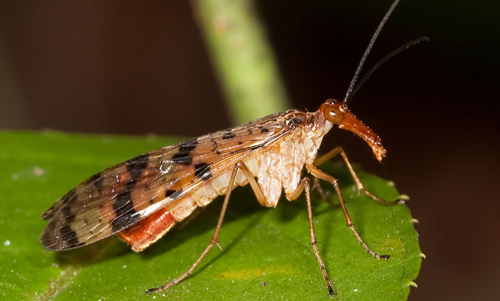This image features a close-up view of a flying insect perched on a large, green leaf, resembling an aloe plant. The insect has a distinct cream-colored body with a reddish end to its tail, and its wings are transparent with an amber hue and black stripes. Its head is particularly notable, with a pointed, red face, jellybean-shaped reddish-brown eyes, and two long black antennas. The insect appears to have six legs, although some descriptions suggest a count of at least five. These legs are thin and spider-like, with upper parts that are whitish in color. In the background, which is blurry and predominantly dark brown to black, there are hints of light green, possibly from another branch or stem extending towards the top. The image captures a mixture of natural elements and varying shades, with the insect's detailed features standing out prominently against the darker backdrop.